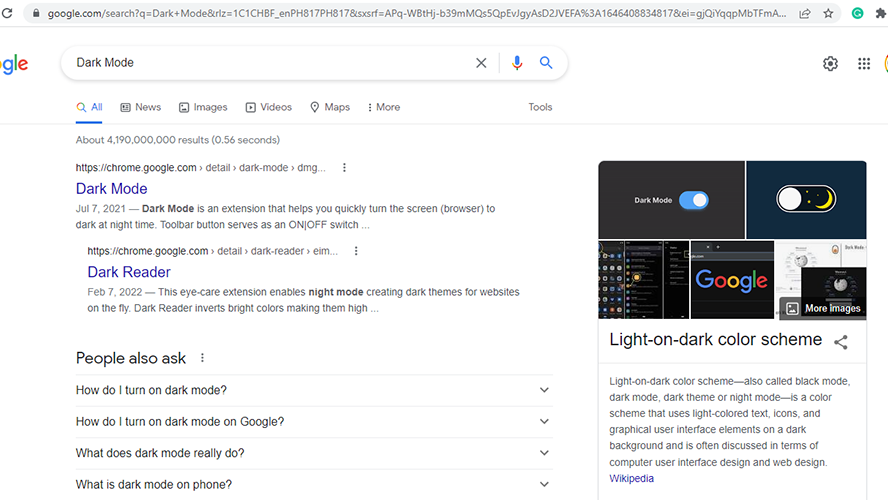The screenshot depicts a Google search results page. The URL, partially visible at the top, confirms the secured connection with a padlock icon and reads "google.com/search." The web page is set to dark mode, as indicated in the search query within the search bar. The search bar contains an "X" to clear the query, a colorful microphone icon for voice search, and a blue magnifying glass icon for initiating the search.

Below the search bar, the available categories for filtering the search results are listed horizontally: All, News, Images, Videos, Maps, More, and Tools, with "All" being underlined to indicate the currently selected category. The search query has yielded approximately 4,190,000,000 results in 0.56 seconds.

The top search result displays a snippet from the URL "https://chrome.google.com" and pertains to the topic of dark mode, specifically a Chrome extension called "Dark Mode," which was detailed on July 7th, 2021. The extension facilitates the transition of browser screens to a dark theme during nighttime, using a toolbar button as an on/off switch.

Following this, the next result mentions "Dark Reader," another browser extension, with the title in blue and additional details in black text. The section "People also ask" includes expandable questions about dark mode such as "How do I turn on dark mode?", "How do I turn on dark mode on Google?", "What does dark mode really do?", and "What is dark mode on a phone?". Each question has a down arrow next to it to reveal further information.

On the right-hand side of the page, there is an illustration featuring a dark mode toggle switch with sun and moon icons, representing the transition between light and dark themes. It includes images comparing a bright and dark screen setting. Accompanying this visual is a paragraph from Wikipedia, explaining the concept of a light-on-dark color scheme.